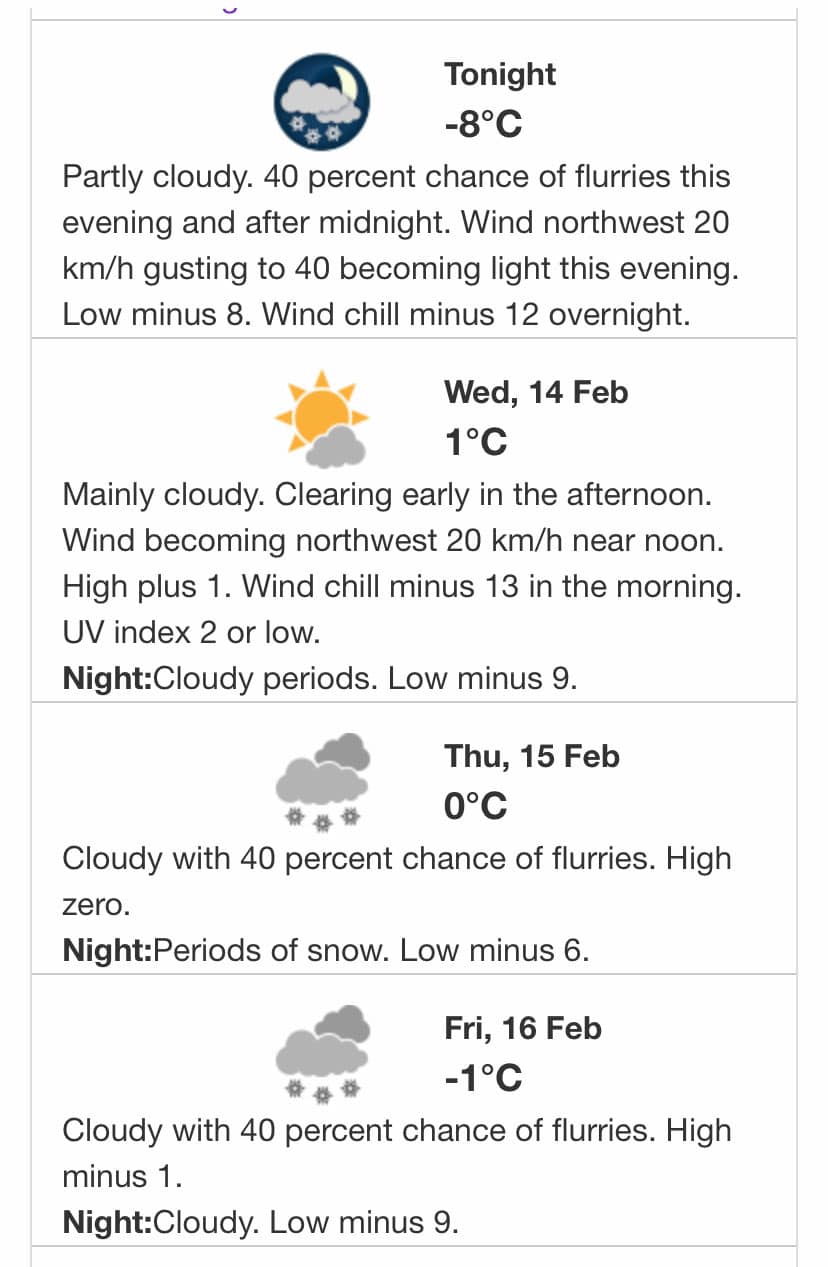This screenshot captures four distinct weather forecast sections from a weather app or website, each dedicated to a different date and arranged vertically against a white background. The topmost section pertains to the current night and indicates a temperature of minus 8 degrees Celsius, accompanied by an icon showing a moon partly obscured by clouds and featuring snowflakes. The second section details the forecast for Wednesday, February 14, with a high of 1 degree Celsius, illustrated by an icon depicting a partly sunny sky. The third section provides the weather for Thursday, February 15, predicting a temperature of 0 degrees Celsius and showing an icon of clouds with snowflakes, indicating potential snowfall. The final section forecasts the weather for Friday, February 16, expecting a temperature of minus 1 degree Celsius, again featuring an icon of clouds with snowflakes. Each section has the day and date displayed on the top right with the corresponding weather icon on the top left, followed by the expected temperature below it.